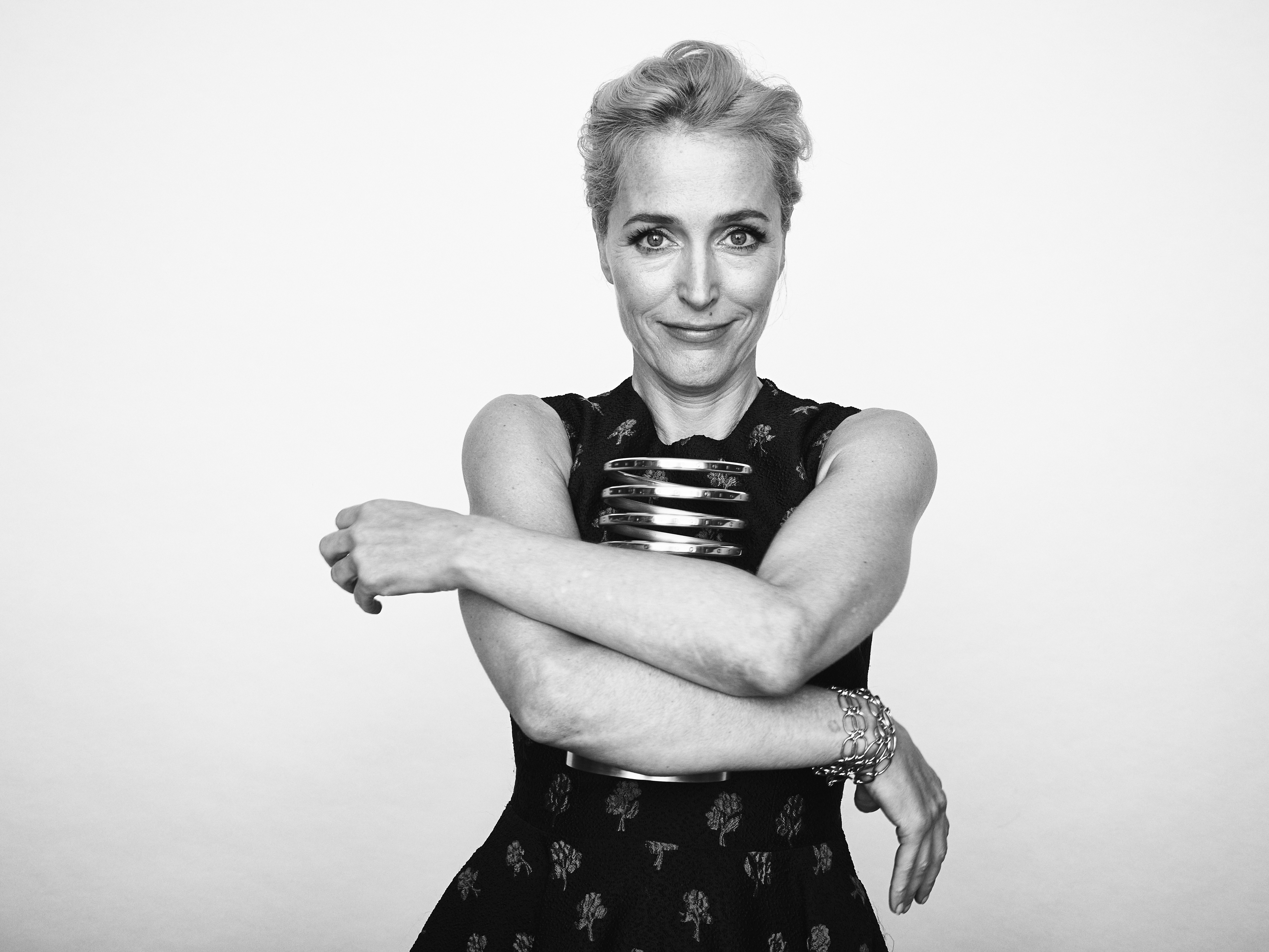This is a black-and-white photograph of a woman with short hair in a pixie cut, detailed to appear either blonde or gray due to the monochromatic filter. She is captured from the waist up, with a modern aesthetic given a vintage touch through lighting and shading effects that cast subtle shadows in the corners, enhancing focus on her figure against an off-white background. The woman, likely in her 50s, wears a sleeveless black dress adorned with a distinctive metallic design down the front, possibly featuring silver flowers and clasps. She holds her arms slightly crossed in front of her, showcasing multiple metallic, circular bracelets on her left wrist. Her face, framed by her short hair, displays a warm smile directed straight at the camera. Enhanced by professional lighting, her makeup is visible, highlighting her mascara and lip gloss, adding to the detailed texture and overall timeless quality of the portrait.